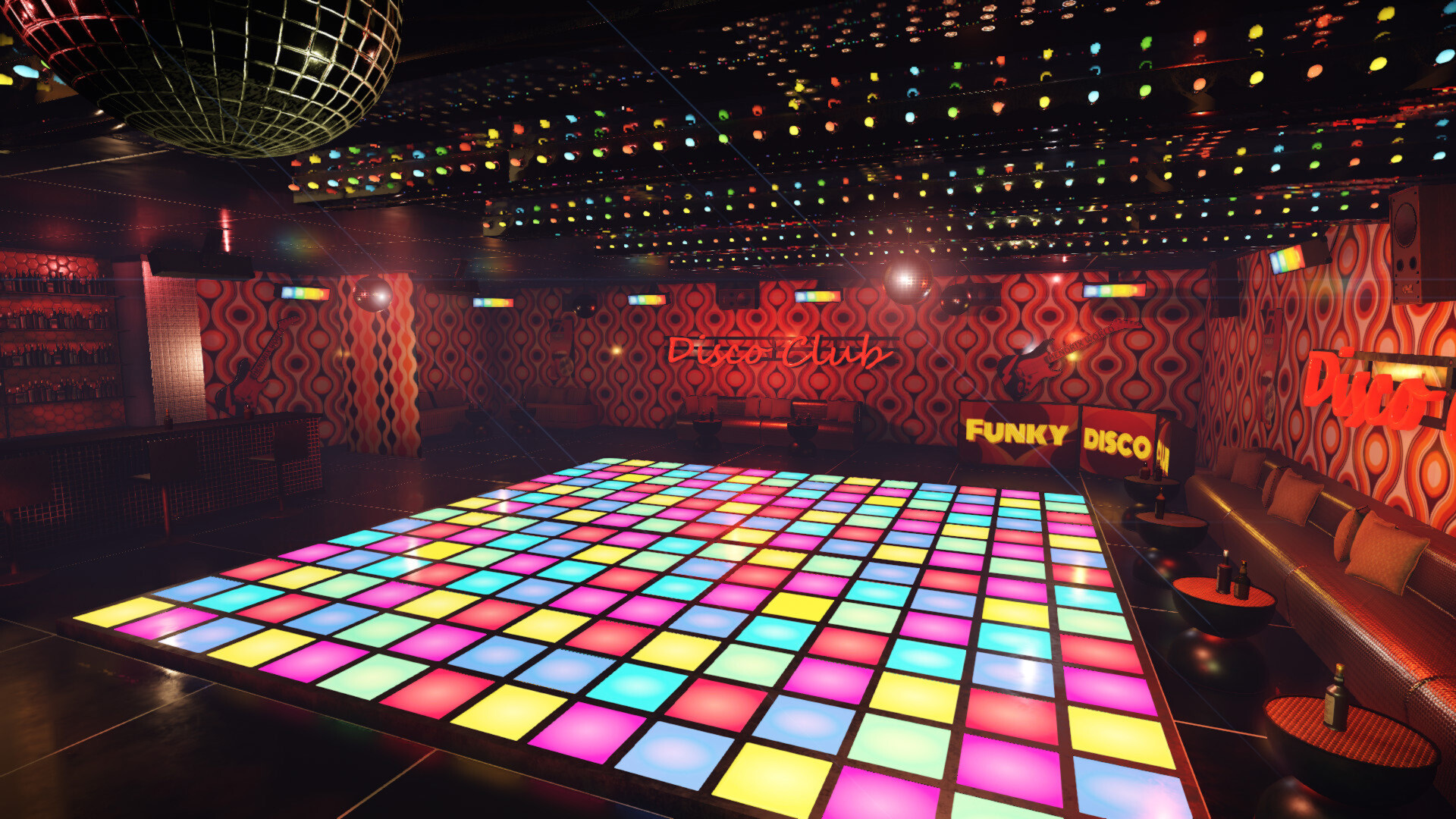The image features an empty disco dance floor within a vividly themed nightclub. At the center, a multi-colored floor made of symmetrical squares in hues of pink, light green, blue, red, and various yellows dominates the scene, with its colors reflecting off the ceiling. The overall ambiance is framed by red geometric print walls, enhancing the party atmosphere. On the right side, a sequence of couches lines the wall, with three small circular tables in front. The first table holds one bottle, the second two, and the third one, possibly beer bottles. A 70s lava lamp-style design extends along the right wall towards the back. The rear wall prominently displays neon signs reading "Disco Club" and "Funky Disco" in bright lights. Above on the left side, a large disco ball with gold emblems and art lighting, representing a globe, hangs from the ceiling. The bar, stocked with bottles on shelves, is located on the left side of the room, contributing to the vibrant décor. Additionally, a funky disco TV screen reflection adds a finishing touch to the overall dazzling setup.